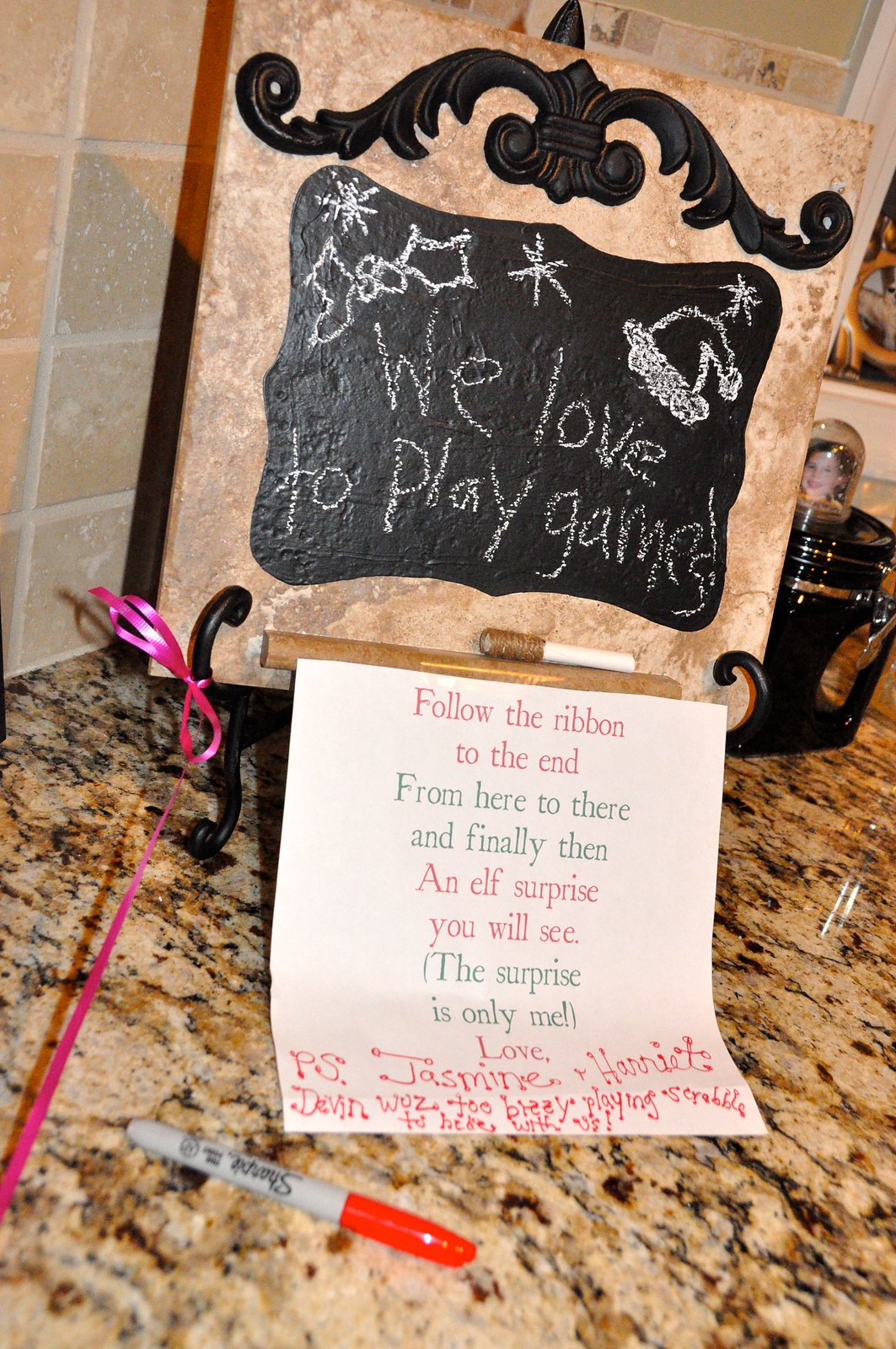The image depicts a charming holiday-themed plaque designed to resemble a small chalkboard, positioned on a black stand on a marble kitchen countertop. Situated against a reddish-brown tiled wall, the plaque features festive chalk drawings of a Santa hat and holly leaves with berries. Across the chalkboard, written in what appears to be a child's handwriting, are the words "We love to play games." The top part of the plaque is adorned with an embossed floral metal design. Below the chalkboard, a piece of paper bearing a playful message is attached. The note reads: "Follow the ribbon to the end, from here to there, and finally then, an elf surprise you will see. The surprise is only me. Love P.S. Jasmine and Harriet. Devin was too busy playing Scrabble to be here with us." A pink ribbon is tied to the stand and extends out of the frame, indicating it may be part of a game, possibly an Elf on the Shelf activity. A gray Sharpie with a red cap rests on the marble countertop, while in the background, a photograph of a young girl is visible to the right of the chalkboard.